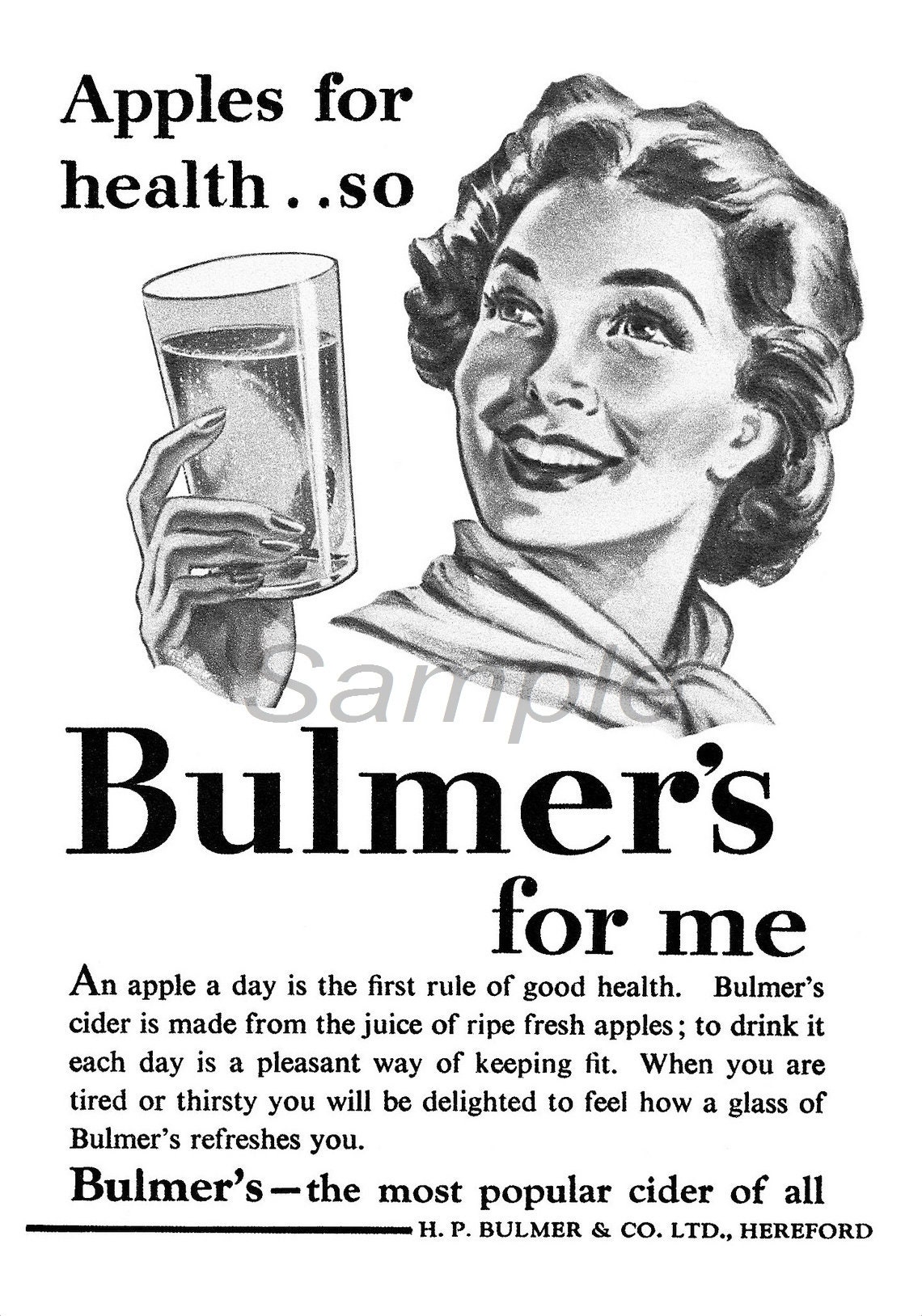This vintage black-and-white advertisement, likely from the 1930s or 1940s, promotes Bulmers cider as a healthful drink. The ad features a cartoon illustration of a smiling woman with curly hair, holding up a clear glass of cider. The headline reads, "Apples for Health... so Bulmers for me." Below the illustration, the text states, "An apple a day is the first rule of good health. Bulmers cider is made from the juice of ripe fresh apples. To drink it each day is a pleasant way of keeping fit. When you're tired or thirsty, you will be delighted to feel how a glass of Bulmers refreshes you." The advertisement claims Bulmers as the most popular cider and notes it is produced by H.P. Bulmer and Company Limited in Hereford.